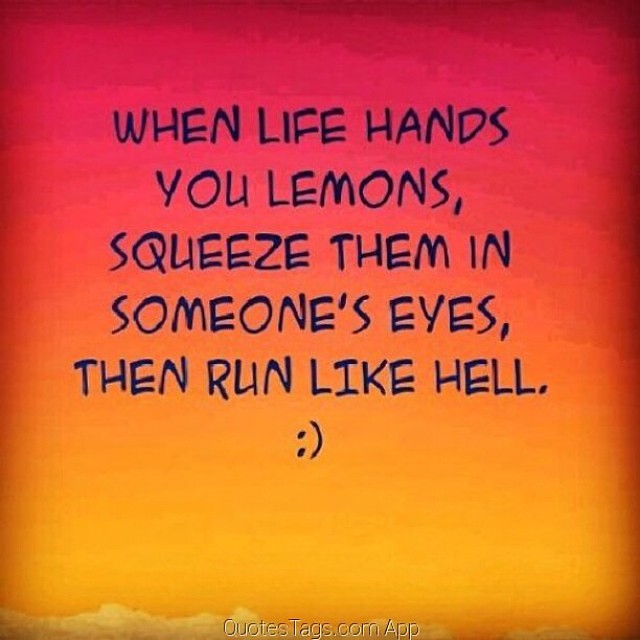The image features a humorous quote set against a striking backdrop of a sunset gradient, transitioning from red at the top, to orange in the middle, and finally to a bright yellow at the bottom. The bottom of the image includes a tan or beige band displaying the text "QuotesTag.com app" in white. The quote itself reads, "When life hands you lemons, squeeze them in someone's eye, then run like hell," followed by a sideways smiley face. The quote text is presented in black, aiming to lighten the mood with its humorous and cheeky advice, characteristic of the content found on QuotesTag.com.